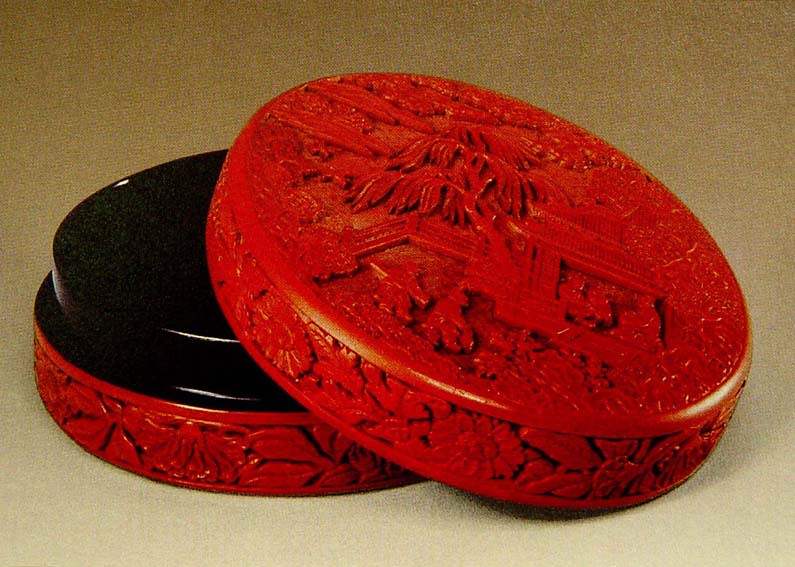This color photograph captures a meticulously posed, indoor scene featuring a beautifully carved, round makeup case that bears a distinctive, ornamental quality suggesting it might be an ancient Chinese artifact, possibly from the Ming Dynasty. The case, which appears to be made of wood with a rich, reddish hue, showcases intricate carvings on both its lid and base. The carvings depict detailed scenes with people, trees, temples, and possibly clouds, enveloped by floral motifs of flowers and leaves. The case unscrews to reveal a black interior, presumably where the makeup is stored, adding to the elegance and historic allure of the piece. The case sits on a textured whitish-brownish table or countertop, further highlighting its intricate and antique appearance.